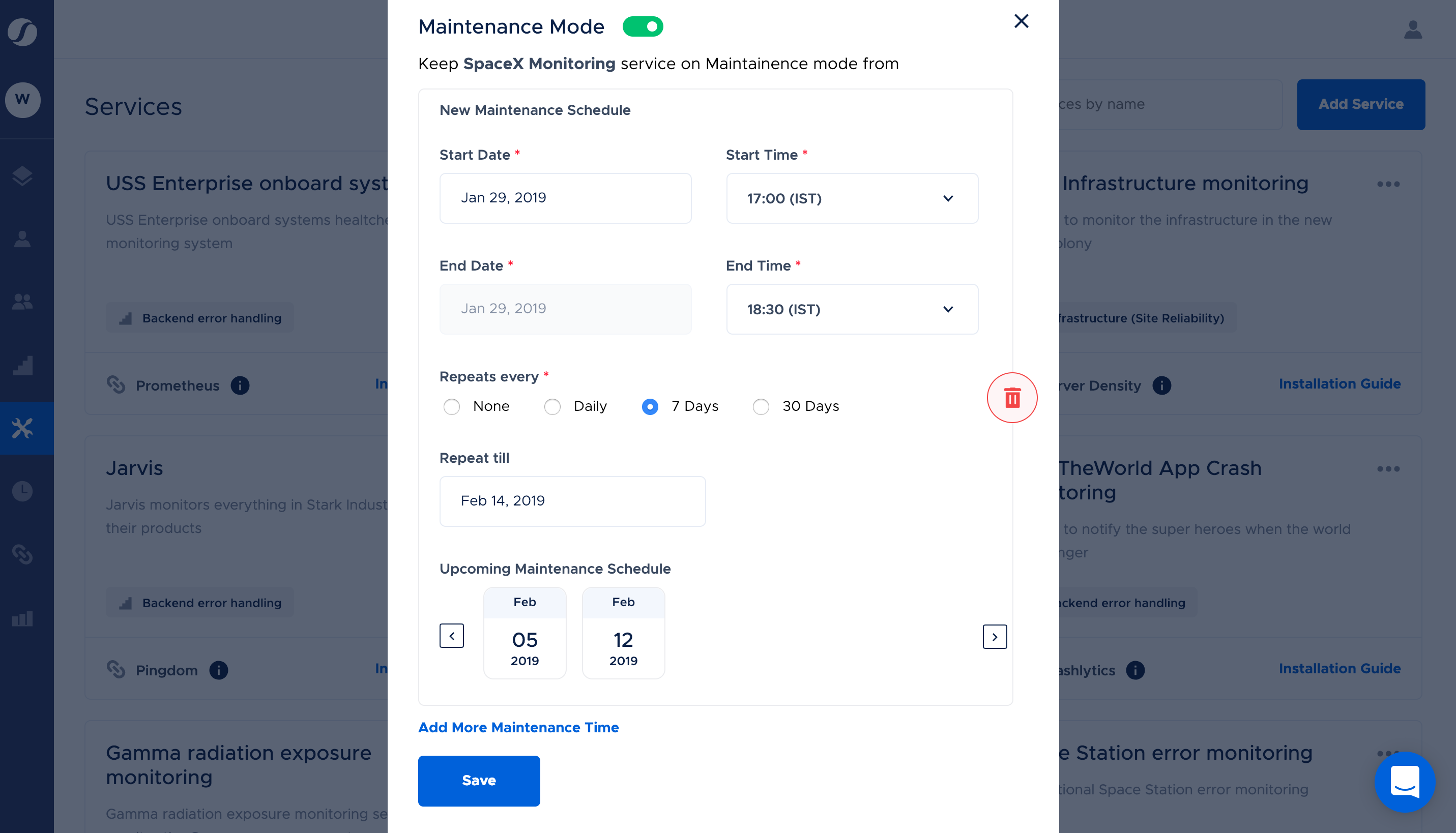The image is a detailed desktop screenshot that does not display the web address, browser, or operating system. On the far left, a grayscale sidebar features various icons: a yin-yang symbol, a circle with a "W," documents, a single person, two people, stairs, a wrench and screwdriver (highlighted in blue), a clock, a chain (representing a hyperlink), and a bar graph. These icons are partially obscured by an overlapping pop-up window.

The left section, slightly visible behind the pop-up, lists several items:
- Services
- US Enterprise Onboard Systems Health Monitoring System
- Backend Error Handling
- Prometheus with an info icon
- Jarvis monitors everything in Stark Industry, their products
- Backend Error Handling (duplicate)
- Pingdom
- Gamma Radiation Exposure Monitoring (twice, possibly a duplicate entry)

The central pop-up is titled "Maintenance Mode," which is toggled to "On." The pop-up includes several fields and controls:
- An "X" to close the window
- A directive to "keep SpaceX monitoring service on maintenance mode from new maintenance schedule."
- Required fields indicated with a red asterisk (*)
- Start Date: January 29, 2019
- End Date: January 29, 2019
- Start Time: 1700 IST
- End Time: 1830 IST
- A setting to repeat every seven days, with an option to delete the schedule
- Repeat until February 14, 2019
- Upcoming Maintenance Schedule
    - February 5, 2019
    - February 12, 2019
- Controls to navigate back or forth to view past or future maintenance schedules, add more maintenance time, and save changes

To the right of the pop-up, partially visible text includes:
- Add Service
- Infrastructure Monitoring
- Infrastructure Site Reliability
- Info Installation Guide
- The world app crash, presumably for monitoring
- Backend Error Handling (another occurrence)
- Analytics Installation Guide
- Station Error Monitoring
- Space Station

The software appears to be a comprehensive monitoring and maintenance tool, applicable for real-life systems and, humorously, fictional scenarios from Marvel movies.